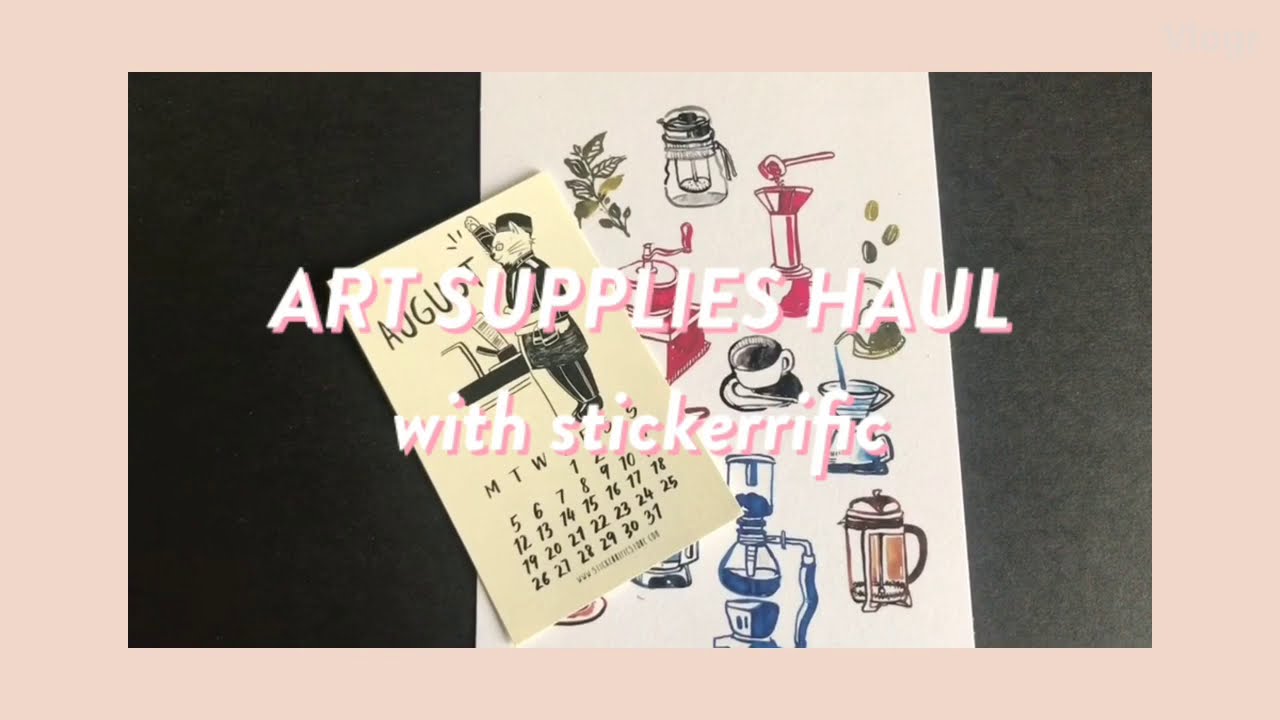The image is a vibrant, detailed screenshot, likely from a YouTube show or podcast, showcasing a variety of artistic and coffee-related elements. At the forefront is a vertically-oriented white sheet of paper filled with detailed hand-drawn illustrations, including leaves, seeds, various coffee makers like a traditional wooden-handled grinder, a French press, and a metal kettle pouring coffee into a blue mug. Notably, a black coffee cup and a plate are also illustrated. To the left of this paper is an August calendar featuring a cartoon cat in a uniform, pushing a tray, with the calendar starting on a Thursday. The image is framed by a light tan-pink border, and the white letters with pink outlines spell out "Art Supplies Haul with Stickerific" prominently in the center. The entire composition lies on a black surface, providing a stark contrast that makes the colorful items pop vividly.